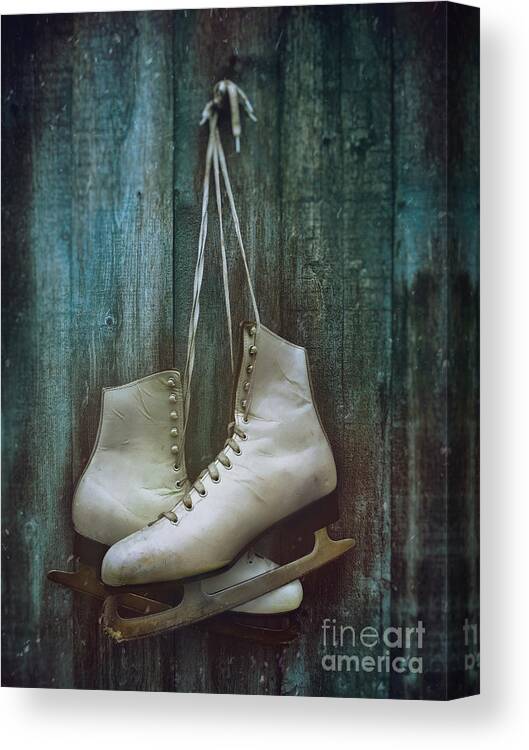The image showcases a piece of artwork displayed on a slightly tilted canvas, which appears to be painted to resemble aged, bluish-green wood. At the center of this canvas, a pair of white ice skates hang by their worn, cracked, and dirty white laces from a hook. The skates, detailed with numerous bends and wrinkles, overlap each other and face opposite directions, with one skate's toe pointing left and the other right. The blades beneath are rusted, showing only sporadic traces of their original silver finish. The overall composition exudes a sense of nostalgic wear and tear. In the bottom right corner of the image, the text "Fine Art America" is prominently displayed, suggesting the origin or distributor of this evocative artwork.